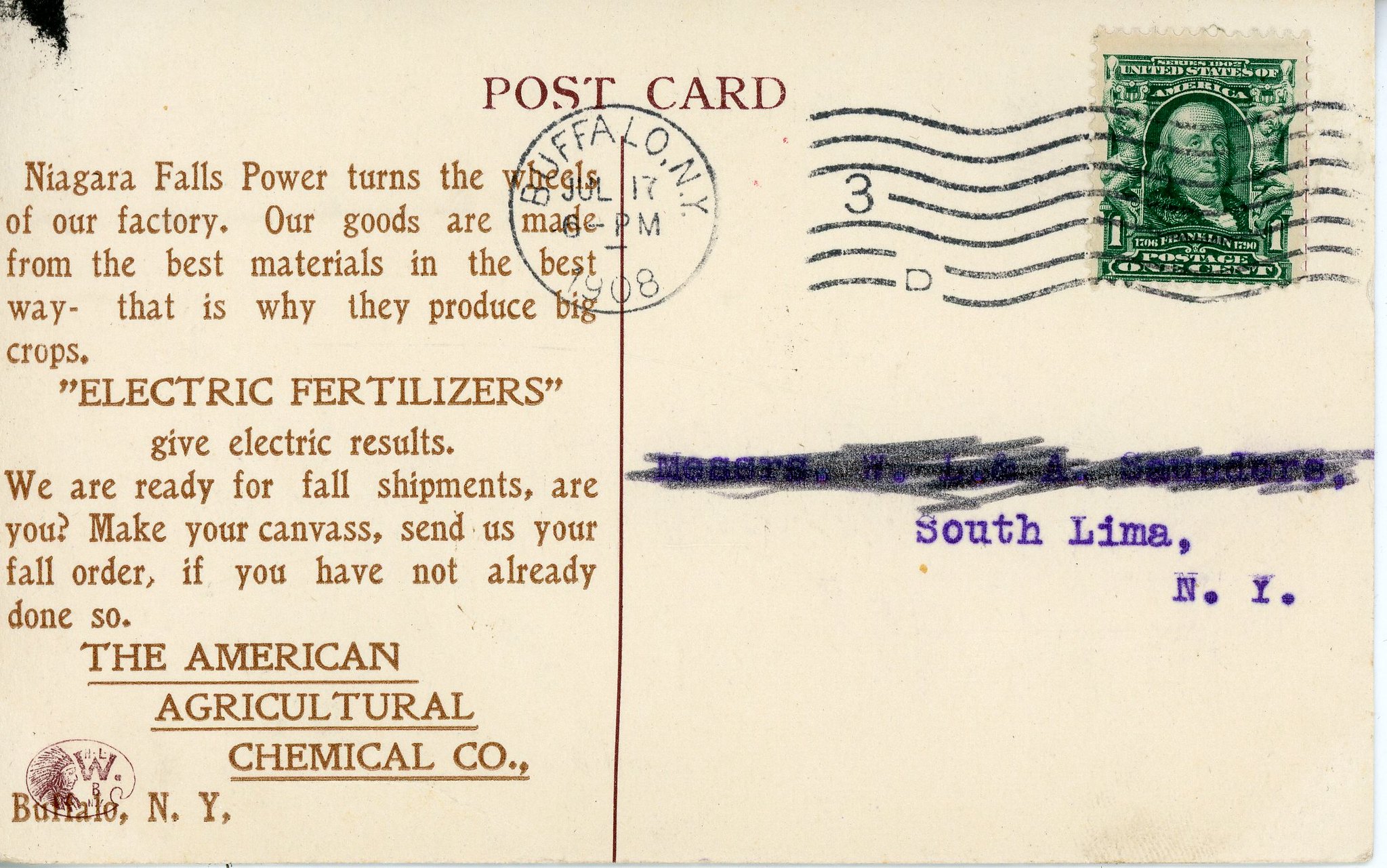This is a close-up photograph of the back of a very old postcard, which appears to be a dark white or yellowish color due to age. The postcard features medium brown print text. In the upper right corner is a green and white United States postage stamp bearing Benjamin Franklin's image and the denomination "one cent." The stamp has been canceled with a black postmark from Buffalo, New York, dated July 17th, 1908, at 6 p.m. Centered at the top of the postcard are the words "Postcard."

On the left-hand side of the postcard, the text reads: "Niagara Falls power turns the wheels of our factory. Our goods are made from the best materials in the best way; that is why they produce big crops. 'Electric fertilizers give electric results.' We are ready for fall shipments. Are you? Make your canvas. Send us your fall order if you have not already done so. The American Agricultural Chemical Company, Buffalo, New York." 

On the right-hand side, where the address would typically be, part of the recipient's name or farm name has been scratched out in black crayon or pencil. However, the town "South Lima, N.Y." remains legible, rendered in purple type print. The combination of these elements provides a fascinating glimpse into early 20th-century communication and advertisement practices.